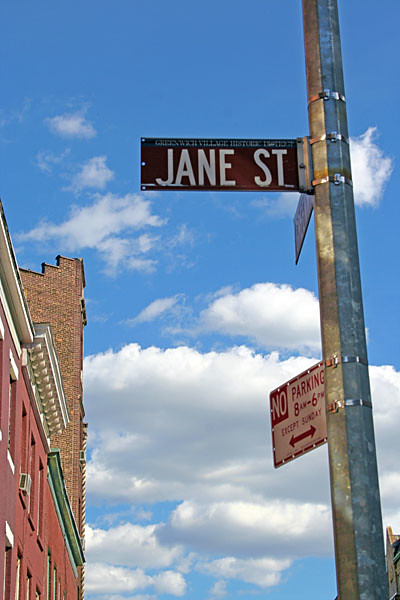The photograph depicts a scene on a picturesque sunny day with a sky painted in a medium bright blue dotted with white, puffy clouds. Among the urban landscape, the second and third stories of a red brick city building can be seen, behind which a taller, brownish brick building looms. On the right-hand side of the image, a metal pole stands, with a street sign extending outward. The sign displays "JANE ST" in white capital letters on a black background. Beneath this, a "NO PARKING" sign in red lettering indicates regulations from 8 AM to 6 PM, except on Sundays, with arrows pointing in both directions. However, the overall composition appears unnatural, suggesting it may be AI-generated. The sky and clouds lack authenticity, the buildings seem artificially placed, and the street sign appears disconnected and incongruent.